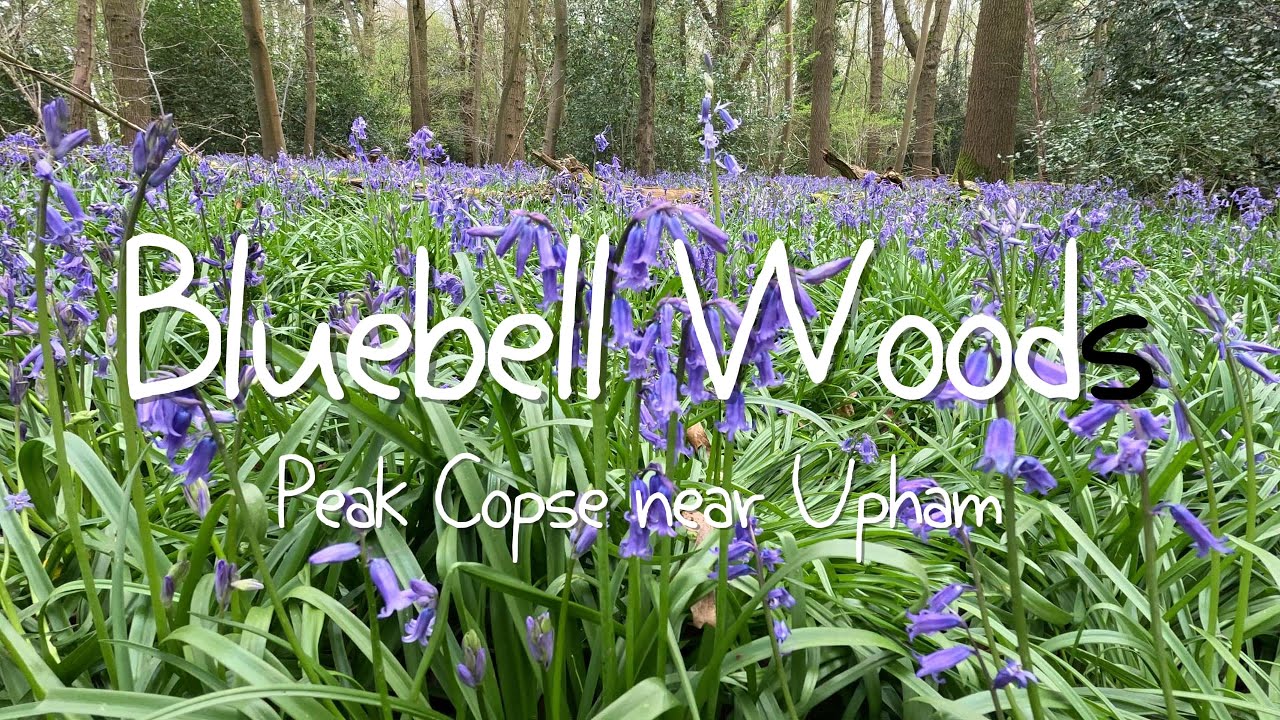The image is a vibrant outdoor photograph taken from a low angle, close to the ground, capturing a sprawling field of tall grasses and lush green bluebell leaves. The bottom and middle portions of the image are dominated by these bluebell flowers, their purple hues scattered throughout the vegetation. In the background, light brown, bare tree trunks rise up, giving way to a dense forest that spans the center of the photo. The sky above suggests a cloudy day, casting a soft, diffused light across the scene. Superimposed on the image are the words "Bluebell Woods" in a white handwritten font with a gray shadow; notably, the "S" in "Woods" is in black. Below this, also in white letters, it reads "Peak Copse near Upham." The image exudes a serene, natural beauty, capturing the understated elegance of the bluebells and their woodland habitat.